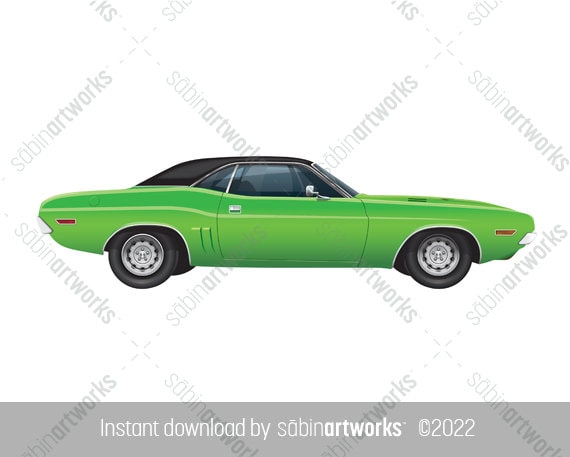In the center of this stock photo, labeled with the watermark "Instant Download by Sabrina Artworks, © 2022" printed in a gray rectangle at the bottom, lies a meticulously detailed drawing of a 1970 Dodge Challenger. The background features a white canvas accentuated by gray zigzagging text that forms a diamond pattern. The green car, showcased from the passenger side at a horizontal alignment, displays a sleek black convertible top and a distinctive white pinstripe running from the rear bumper to the front hood. Additional features include a silver side mirror, silver handles, black tires with silver rims, and two vents located on the rear bumper in front of the right rear tire. The car is a classic two-door coupe, embodying the quintessential design elements of 1970s sports cars.